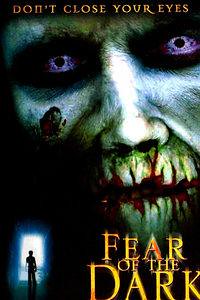This vertical cover illustration, possibly for a book or DVD, predominantly features a terrifying face that merges elements of a ghostly skull and a monster-like zombie. With menacing purple eyes, jagged and bloody teeth, and pale, gruesome flesh, this face dominates the upper portion of the cover. The topmost black text chillingly reads "DON'T CLOSE YOUR EYES." Below the haunting face, in the bottom-left corner, a shadowy silhouette of a person is seen standing in an illuminated doorway, adding a sense of impending doom. The title "FEAR OF THE DARK" is displayed in striking gold capital letters on the bottom right. The image uses a color palette that includes shades of gray, green, red, white, black, blue, and yellow, creating a haunting and foreboding atmosphere.